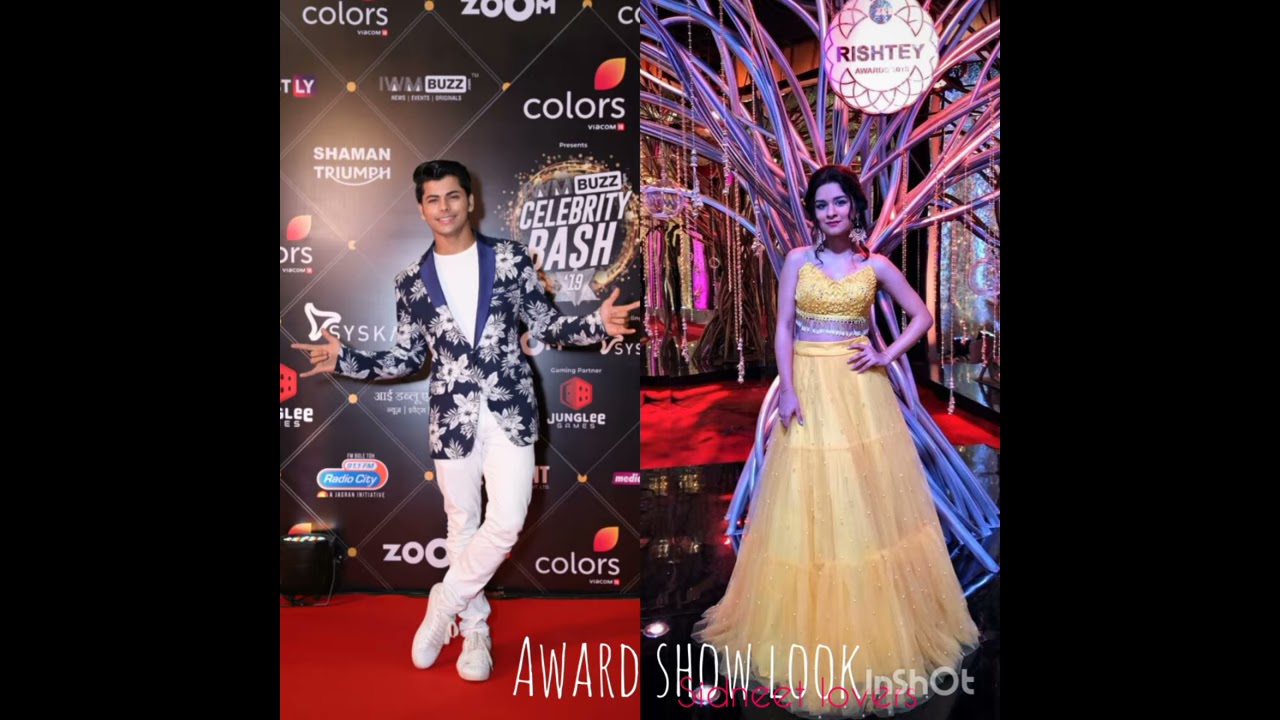The image consists of two distinct photographs framed by broad black bars on the left and right sides. On the left, a man with olive-toned skin and dark brown hair is featured standing on a red carpet at a high-profile event, likely a celebrity bash or award show. He is dressed in a striking floral-patterned blue blazer over a white shirt, paired with white jeans and white sneakers. Behind him, an advertising backdrop lists event sponsors, along with the words "Buzz," "Celebrity Bash 19," and "Jungle Games." The man is making a peculiar hand gesture with his ring and middle fingers down and other fingers pointing outward.

On the right, a woman who also seems to be an actress, possibly from Bollywood, stands elegantly on another red carpet. She is wearing a vibrant, strapless yellow gown that cinches at the waist and flows outwards, complemented by dramatic, dangly earrings. Her dark hair is styled back, and she poses confidently with one hand resting against her body and the other on her hip. The setting behind her features a vivid and elaborate design, reminiscent of a disco or high-class event space. Below both photos, text reads "Award Show Look Sydney Lovers," uniting the two separate images in a cohesive theme of glamorous red carpet appearances.